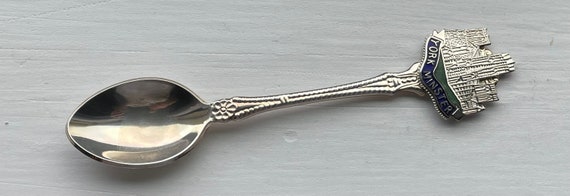This is an image of a collectible silver teaspoon resting on a white wooden surface with a visible grain texture. The spoon is angled, pointing slightly to the bottom left. The spoon’s bowl is smooth and reflective, catching some of the light. The handle features an intricate and embroidered design that includes dots spanning its entire length. At the meeting point of the spoon and handle, there is an embellishment resembling a small flower. Further up the handle, just below an emblem depicting a skyline or cityscape, there’s a mix of green color right above a blue banner. The banner displays "York Minster" in white capital text. The entire image is well-lit, highlighting both the detailed designs on the handle and the reflective surface of the spoon.